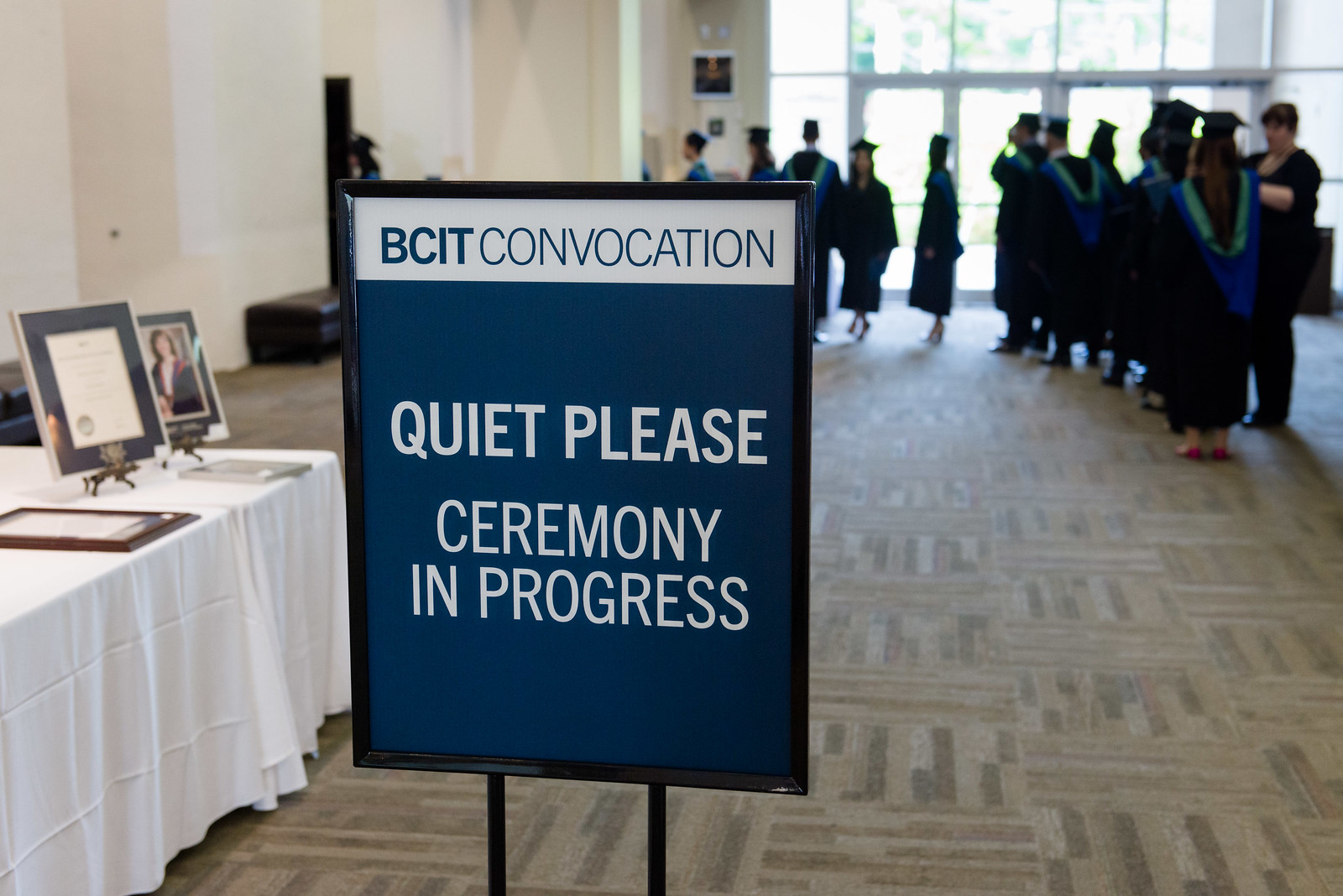The image depicts the entrance to a college graduation ceremony, specifically a BCIT Convocation. Prominently positioned in the foreground is a sign encased in a black metal frame, mounted on poles. The sign features a white ribbon on top with the navy blue letters "BCIT Convocation" and below, a solid blue background with the message "Quiet Please Ceremony in Progress". To the left of the sign, a white table draped with a white cloth holds several indistinct picture frames. The floor of this commercial space is a gray carpet. The setting is bright, with light streaming in through a set of four glass double doors, which are flanked by large glass windows. In the distance, a line of college-age students wearing black gowns adorned with blue and green, and black caps, are visible. One lady seems to be conversing with a student. The surrounding walls are white, and there's a leather couch against one wall, adding to the room's formal yet comfortable atmosphere.